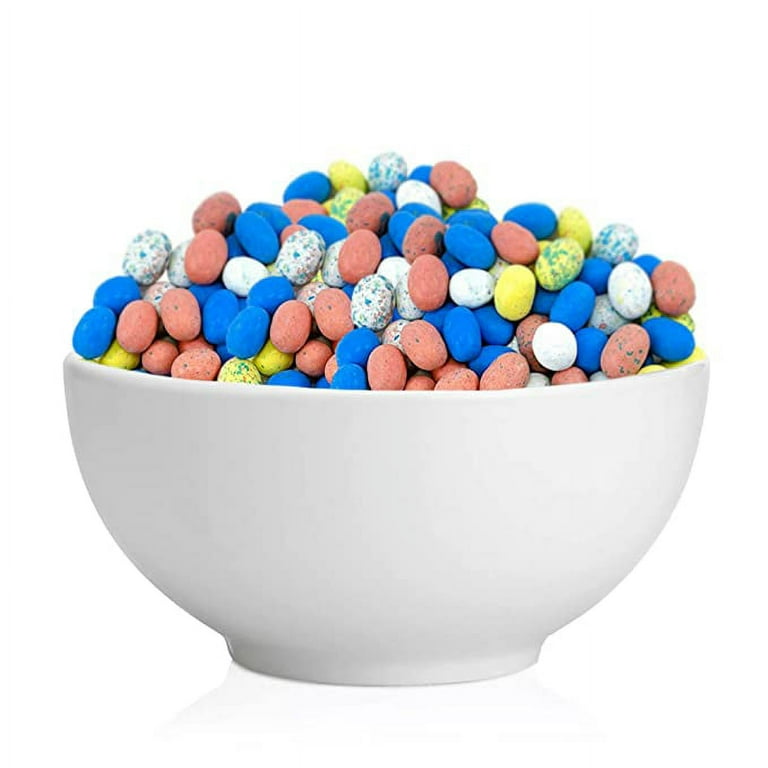The photograph showcases a square image with equal-length sides, featuring a white porcelain bowl brimming with an assortment of spherical candies. The bowl, resting on a reflective white surface, casts a subtle drop shadow and is designed in a widening, half-moon shape. The bowl is filled to the top with vibrant, matte-textured candies that resemble Easter malted eggs or dusty jelly beans. The candies come in a variety of colors: dark blue, pink, yellow with green spots, white with green spots, as well as speckled variations. Specifically, there are bright blue ones, yellow ones with blue specks, plain white ones, and white ones with splatters of color. The background is entirely white, making the colorful array of candies the focal point of the image.